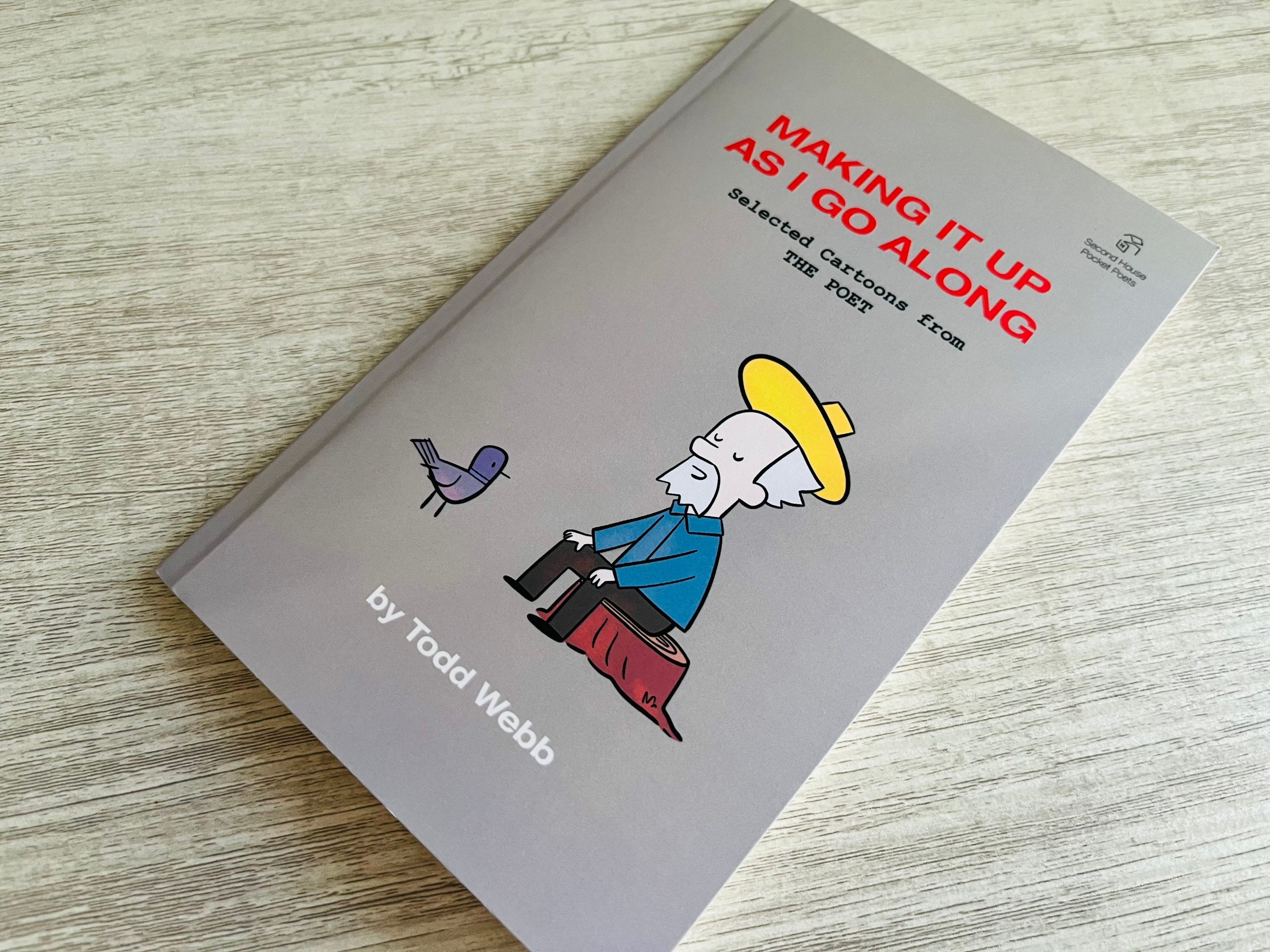The image is a color photograph taken in landscape orientation, capturing a small book positioned on a light gray surface that simulates wood grain. The book is placed diagonally, with its top pointing toward the top right corner and its bottom toward the bottom left. The cover of the softcover book is solid gray and features multiple lines of text. At the very top, red text reads, "Making It Up As I Go Along," followed by smaller black text, "Selected Cartoons from the Post." In the upper right corner of the cover, the publisher's mark, "Second House Pocket Poets," is displayed. 

The center of the cover showcases a detailed line drawing of a bearded man with white hair. He is depicted sitting on a brown tree stump, facing to the left with his eyes closed and hands resting on his knees. The man wears a broad-brimmed yellow hat, a blue long-sleeved shirt, and black pants. In front of him on the ground is a small blue bird looking up at him. At the bottom of the cover, white text reads, "By Todd Webb." 

The lighting in the photograph comes from the center-right, illuminating the book and enhancing the gray and wood-grain textures of the background.